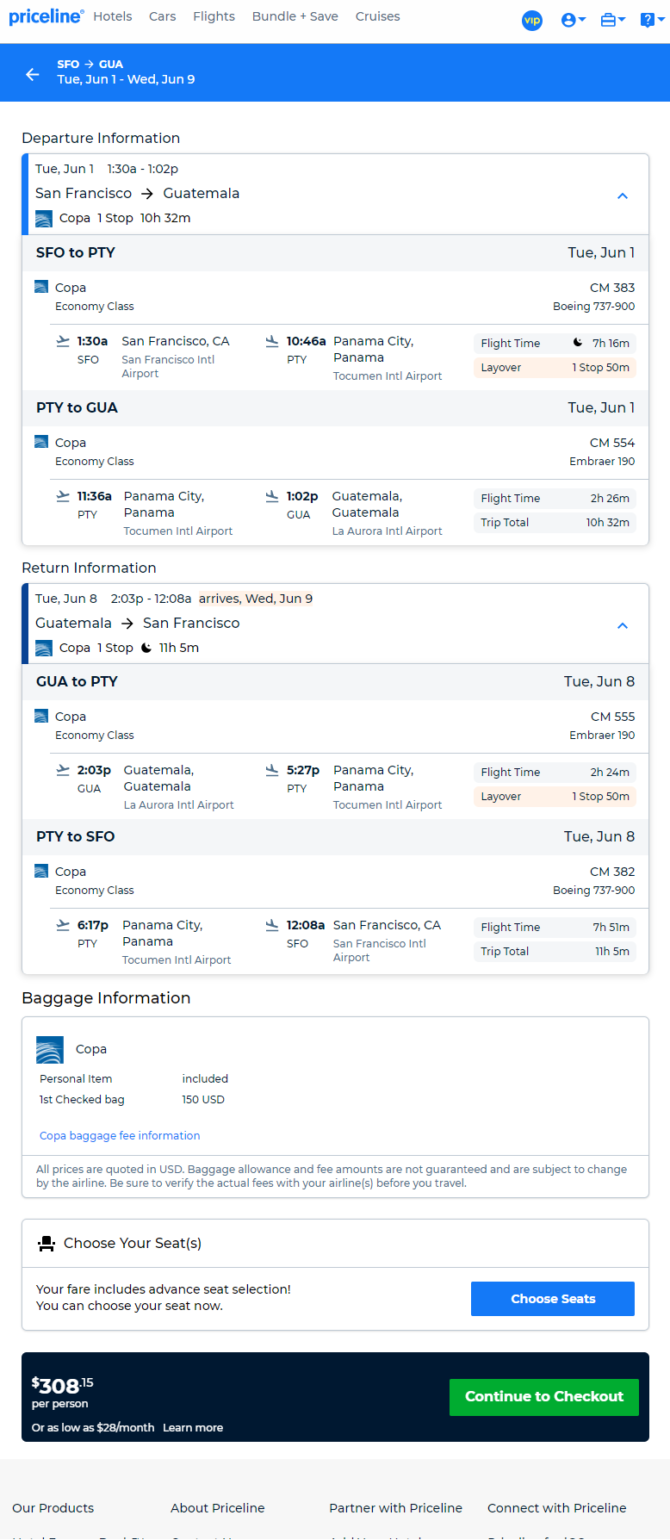The image features a flight itinerary interface set against a light blue background at the top. The layout includes a price line and several headings accompanied by small icons. Below these, a bright blue box dominates the screen. This box includes a left arrow and text displaying departure information. On the same blue background, there is a smaller box with a blue line on the left side showing the route from San Francisco (SFO) to Guatemala (GUA) via Panama City (PTY). 

The details for the flight appear in various sections, with some information contained in tiny blue boxes. The first segment features the flight from SFO to PTY on Tuesday, June 1st. This section also includes an up arrow, some additional information, a little airplane icon, and a mix of blue and pink boxes that segregate different parts of the details. 

Following this, another blue section outlines the second leg of the journey from PTY to GUA, further divided into two white boxes. These white boxes contain tiny blue boxes with flight information and return flight details.

Subsequently, there is a white box with a blue line down the left side detailing the return journey from GUA to PTY, also including a tiny blue box. Moving right, more information is displayed within blue and pink boxes for the flight from PTY to SFO on Tuesday, June 8th. 

Finally, the itinerary includes baggage details and a prompt to choose seats, marked by a blue button. At the bottom, a prominent black box shows the price per person at $308, accompanied by a green button labeled "Continue to Checkout." Additional words are visible at the bottom within the light blue section of the interface.